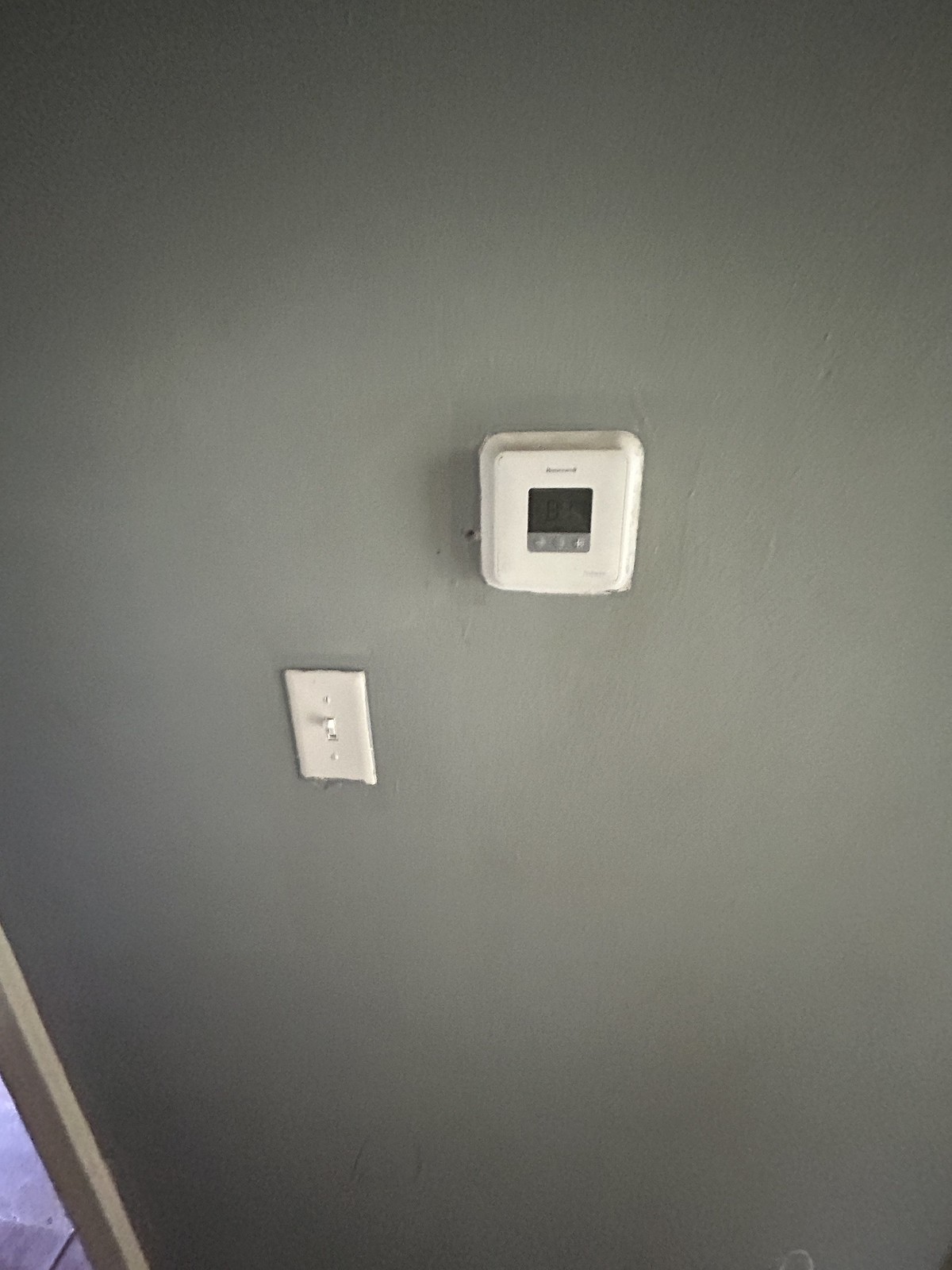The image predominantly features a wall, occupying approximately 90-95% of the frame. The wall is constructed of wood and painted a darker gray shade, although the paint appears uneven, particularly in the upper section where some splotches are visible. At the bottom left corner of the image, a segment of light gray cement flooring is visible, enhancing the simplicity of the scene. Adjacent to the flooring, a light gray vertical post runs upwards along the border of the wall.

Two objects are affixed to the wall. Situated towards the middle right of the image is a square device with a white background. This device features a smaller square section in its center, displaying the number "84" through a glass window, along with a gray rectangle below containing three indistinguishable buttons.

The second object, positioned in the middle bottom left of the full image, is a light switch. The light switch has a vertical rectangular form, oriented with the switch itself in the 'up' position. Accompanying the switch are two screws aligned vertically below it.